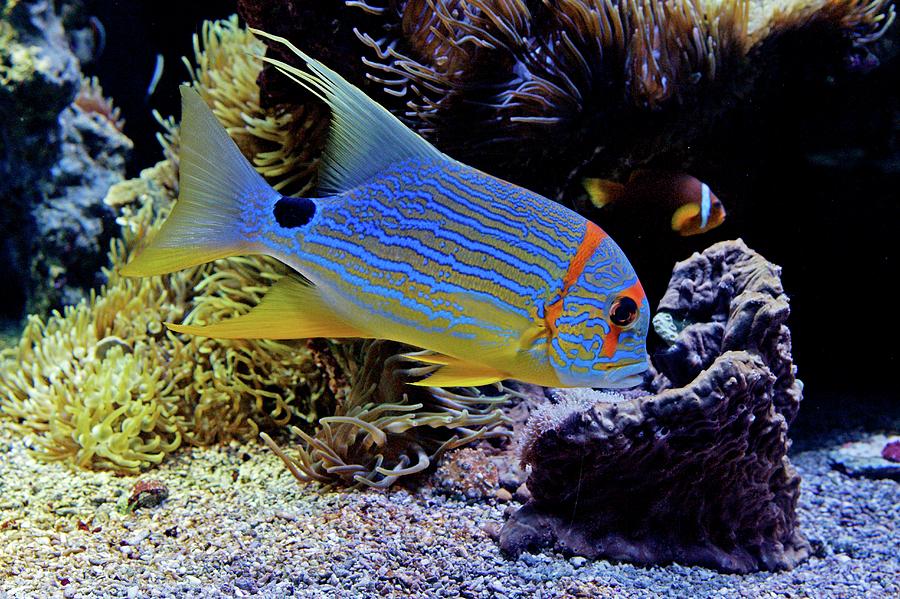This vibrant underwater image portrays a striking sky blue and yellow angelfish swimming gracefully in a saltwater environment. The angelfish, positioned with its head to the right and tail slightly elevated to the left, displays a fascinating pattern of blue and yellow horizontal stripes along its body. Notably, a bright orange vertical stripe decorates the area near its eye and gill, while its lower fins and belly exhibit a more pronounced yellow hue. A distinctive black spot is visible near the base of its tail. The aquatic scene is enriched by a variety of elements: a yellow plant to the left of the fish, purplish coral with indigo tips on the right, and colorful purplish rocks in the foreground. Adding to the marine ambiance, floating sea anemones and a nearby clownfish populate the backdrop, enhancing the photograph's depth and richness.